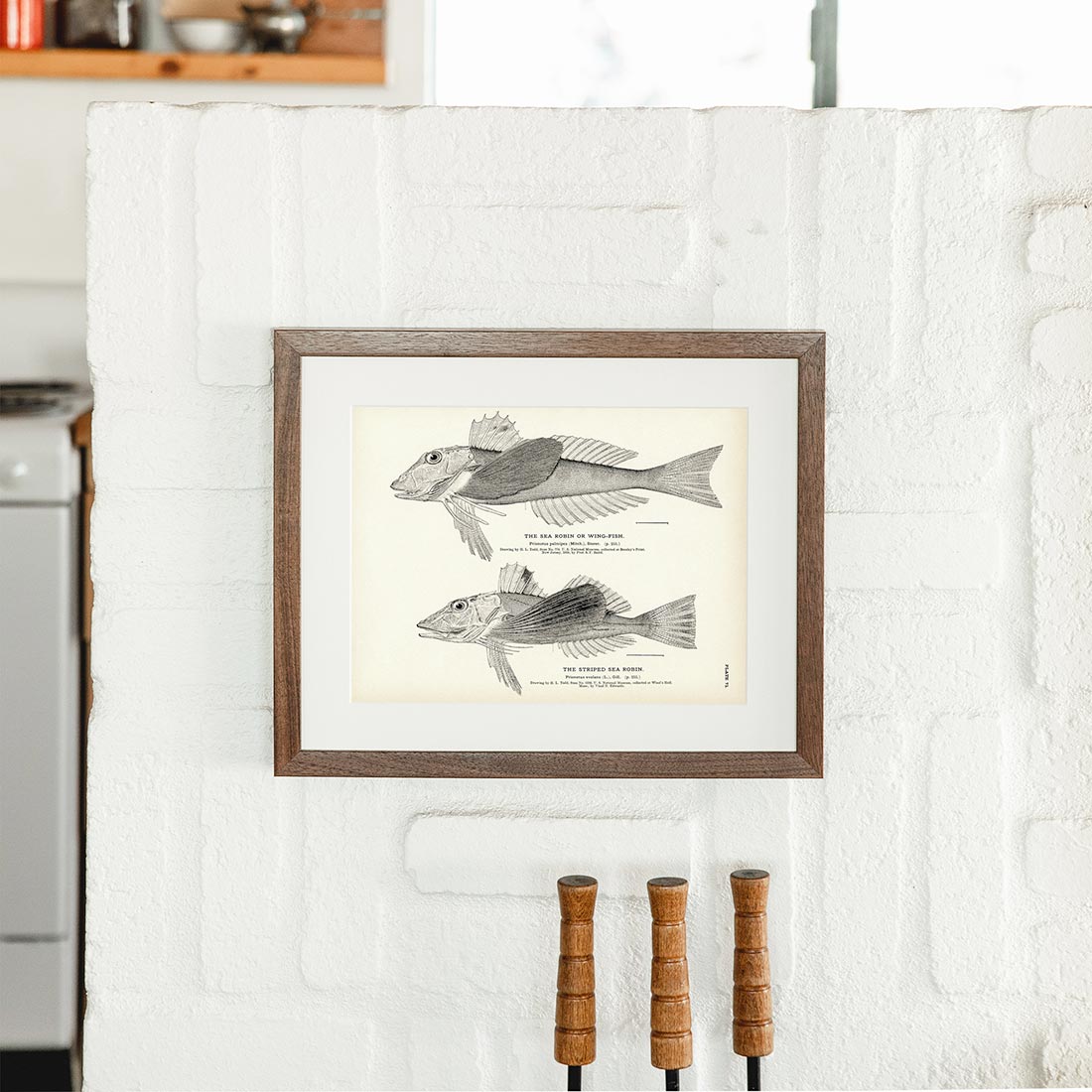The photograph captures an interior scene showcasing a section of a white-painted brick wall, prominently featuring a framed illustration of two meticulously detailed black and white fish, evocative of those found in old nature or scientific journals. The frame is wooden, complementing the neutral-toned decor. Each fish is labeled—though the text is largely unreadable—with visible names suggesting the species as different types of sea robins, known for their distinctive, almost leg-like appendages. The artwork hangs above what appears to be a fireplace, as indicated by the partial view of three fire poker handles made of wood and iron at the bottom of the image. In the distant background, a white stove is visible, along with a brief glimpse of a wooden shelf or cabinet, partially stocked with kitchenware, maintaining the predominant white and wooden aesthetic of the space. This photograph could easily feature in an interior design magazine or website, highlighting the blend of scientific art and functional home décor.